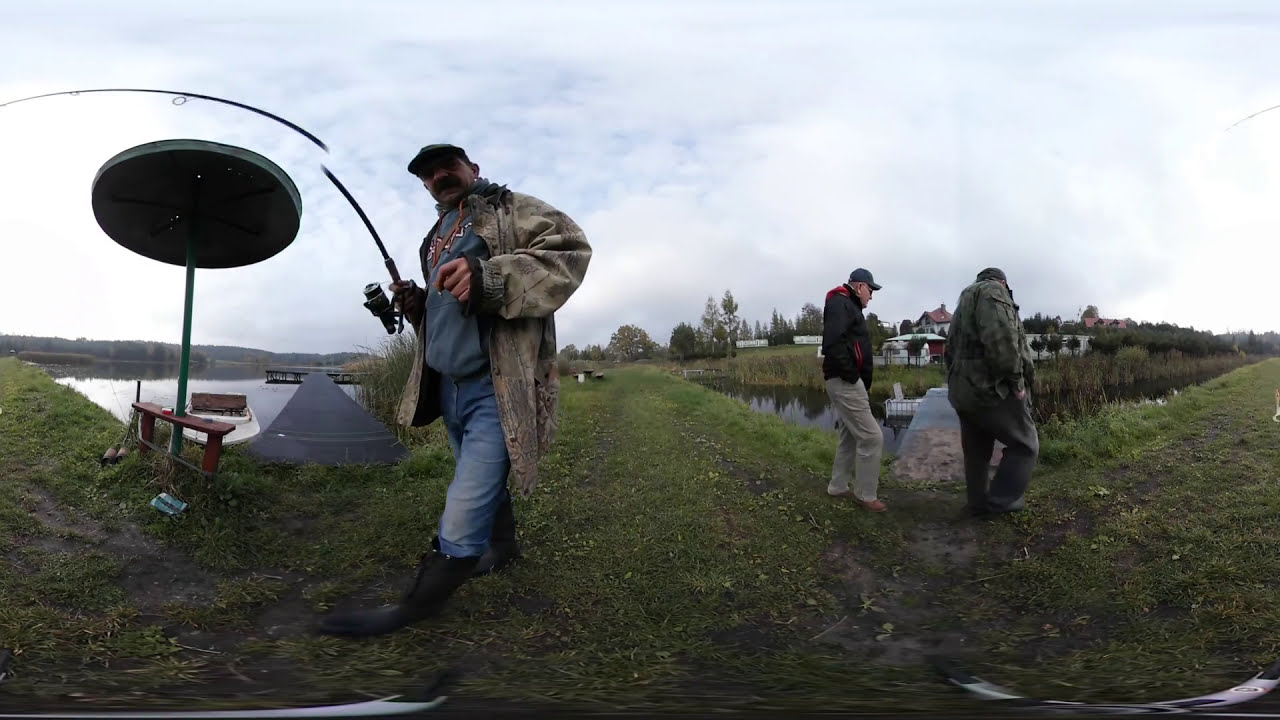Three men, appearing to be middle-aged and older, are outside in a countryside setting, standing on grass interspersed with patches of mud. The central figure, heading towards the left, wears a military-style gray-green jacket over a gray sweatshirt, blue jeans, tall black boots, and a ball cap. He holds a possibly broken fishing pole in his right hand. To his left, the two other men are walking separately: one wears a dark jacket, ball cap, and dark pants, while the other has a dark jacket, ball cap, and khaki pants. They all seem to be fishermen. The scene features two ponds or lakes, suggesting a fishing area, under an overcast sky with clouds. Additional details include a dock, an umbrella, a brown bench, a nearby building on the right, trees in the background, and a plank near the water, enhancing the rural ambiance.